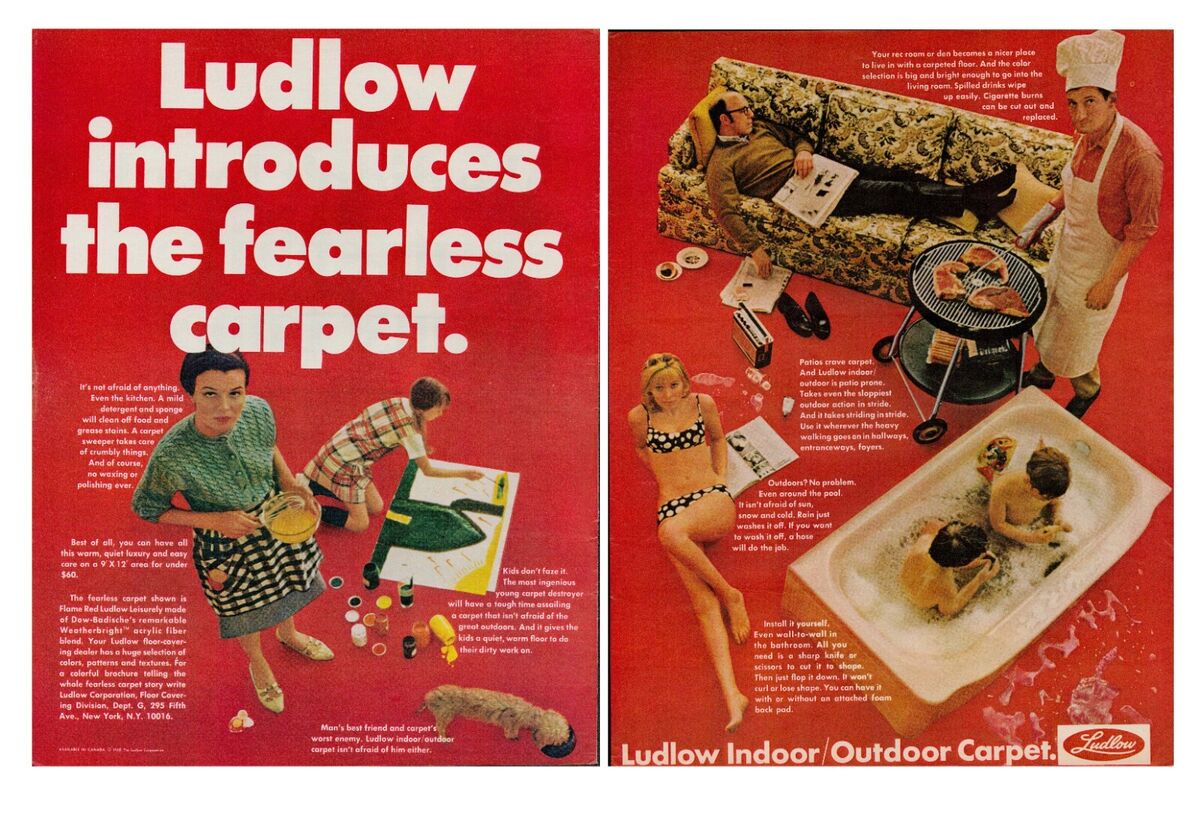This double-page advertisement showcases Ludlow's Fearless Carpet against a vivid red background. On the left page, large white text reads "Ludlow Introduces The Fearless Carpet". Below this, a woman with black hair, dressed in a green button-up cardigan and a black-and-white checkered apron, is beating eggs in a clear, yellow-filled bowl. To her right, a little girl draws on the carpet with her art supplies scattered around. A dog is nearby, eating from a dish. The right page features a man sleeping on a couch at the top, with a man barbecuing below him. A woman in a bathing suit lounges on the carpet to the left. At the bottom, children are seen bathing in a tub placed on the carpet. Both pages are framed by additional descriptive text, emphasizing the versatility and durability of the Ludlow Indoor Outdoor Carpet.